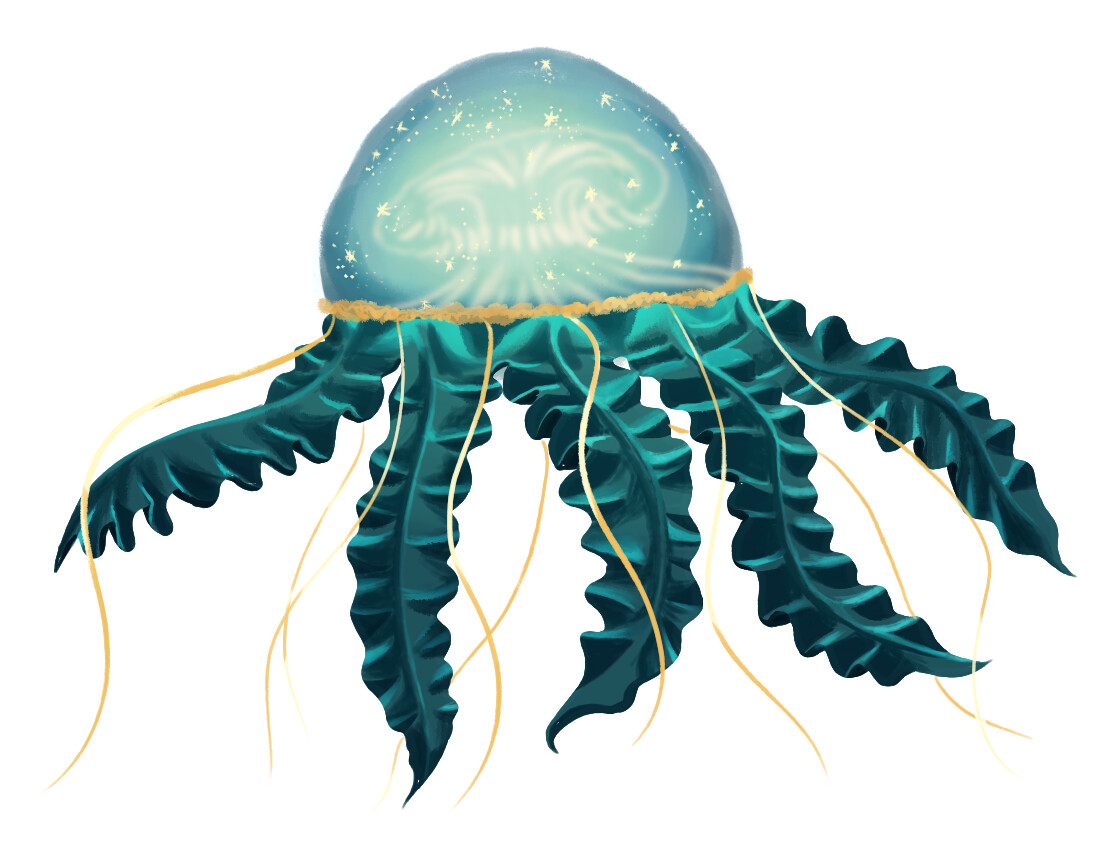This digital illustration features a stylized jellyfish with a distinctly cartoonish quality. The jellyfish's semi-spherical head is centrally positioned against a white background, boasting a gradient of teal hues—darker on the edges and much lighter in the center, giving it a shiny appearance. Accentuating the head is a golden band along its lower edge. Below the head, five elongated, dark teal tentacles, reminiscent of ruffled leaves, extend sporadically outwards. Additionally, numerous thinner, wavy golden tendrils emanate from the area near the tentacles, adding a whimsical touch to the illustration. The overall image blends elements of marine life with a fun, imaginative twist.